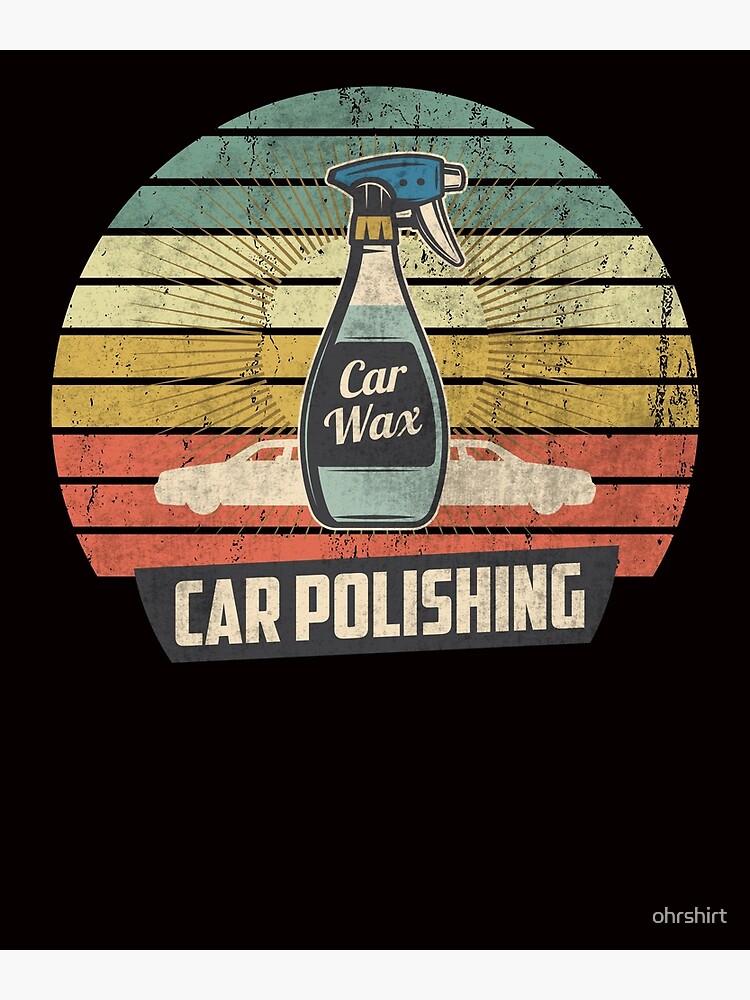The poster showcases a detailed design against a black background, dominated by a central transparent spray bottle with a blue head filled with blue liquid. Midway up the bottle, a black sticker reads "CAR WAX" in white ink. Surrounding the bottle, two white silhouettes of car fronts emerge from either side. Above this central image, an off-centered circular shape is adorned with vibrant horizontal stripes: three red at the bottom, followed by two shades of brown, then two shades of yellow, topped with three blue rows. At the circle's base, a blue sign with white text boldly declares "CAR POLISHING." The bottom right corner of the poster discreetly features the text "OHR SHIRTS" in white. The entire layout suggests a theme of automotive care, seamlessly integrating colorful elements and sleek design features.